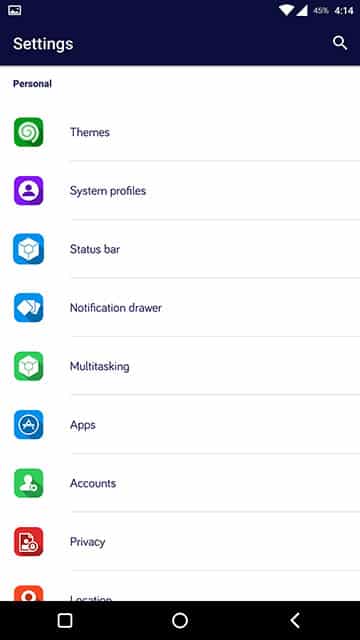This is a mobile screenshot of a settings panel on a cell phone. The interface begins with a dark blue banner at the top, displaying the word "Settings" in large white font, positioned in the bottom-left corner. Beneath this banner, the body of the app has a white background. At the top-left corner of this section, the word "Personal" is written in small black letters.

The settings options are organized in a vertical list, with each setting separated by a thin gray line. The icons for each setting are aligned along the far left side of the panel. The first setting listed is "Themes," accompanied by a green square icon to its left. Below "Themes," in sequence, are the settings for "System profiles," "Status bar," "Notification drawer," "Multitasking," "Apps," "Accounts," "Privacy," and finally "Location." The "Location" setting is positioned about halfway down the screen, indicating that additional settings can be viewed by scrolling further down.